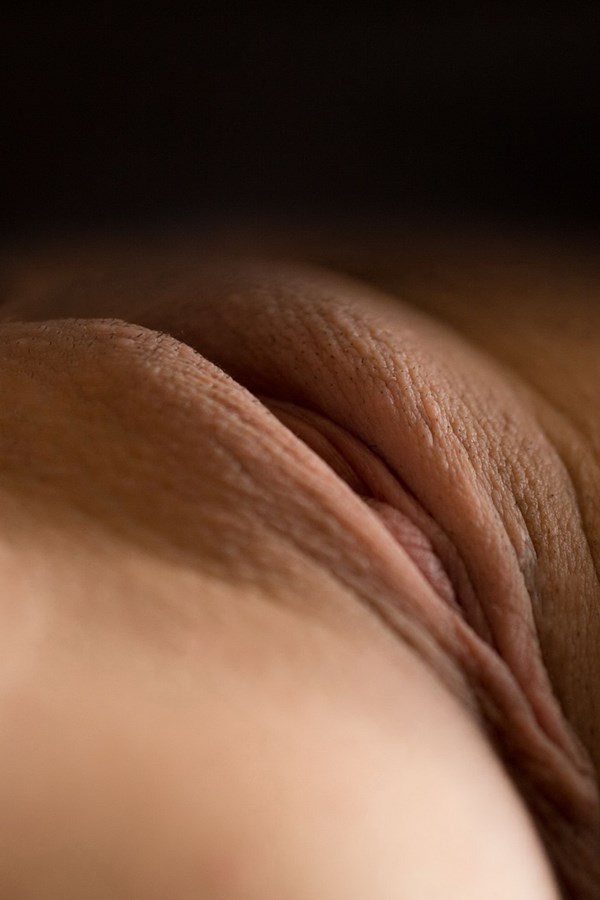This is an extreme close-up image primarily showing skin that appears to belong to a part of a human body. The top third of the image is dark and shadowed, obscuring much detail. As the image moves downward, the fair, hairless skin becomes more illuminated and visible. The smooth texture of the skin is evident, though a section in the middle appears wrinkled or folded, suggesting it could be an eyelid or another body part such as the vulva. The exact identification of the body part remains ambiguous due to the proximity of the shot and lack of additional contextual clues.